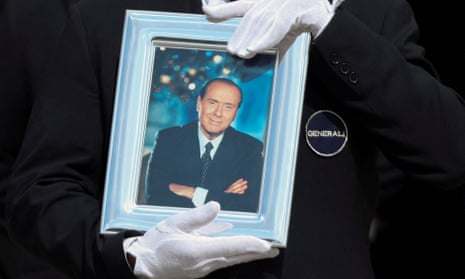The image depicts a photograph framed in a light blue frame with a subtle ridged design. The photograph within the frame captures a man in his 50s or 60s, dressed in a buttoned-up black suit paired with a black tie and a white dress shirt underneath. The man, a white male, has a high receding hairline and thin, dark hair. He is slightly smiling with a closed mouth, arms crossed in front of him in a somewhat confident pose. 

Holding this framed photograph is a person clad in a black suit, noticeable for the white gloves that they are wearing. The white gloves, stark against the solid black background, draw immediate attention to the frame and its contents. One gloved hand is placed at the top of the frame while the other supports it from the bottom. Additionally, there is a circular insignia or label on the right side of the photograph that reads "general," suggesting either the man in the photo or the individual holding the frame might have a military connection. The overall composition emphasizes the formality and the focal point of the man in the photograph, highlighted against the subdued and dark backdrop.